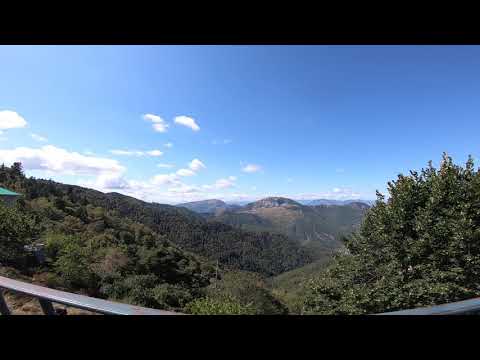This detailed landscape photograph captures the lush, rolling hills and distant mountain ranges from a scenic viewpoint, possibly a balcony. In the foreground, a partially visible metal fence hints at the vantage point. The terrain is a mixture of vibrant greens from trees, bushes, and lush vegetation, interspersed with patches of dried, brown grass indicative of a warm, possibly desert-like climate. The horizon showcases an expansive, clear blue sky accented by a few puffy white clouds, with the sky deepening in blue towards the top of the image. The wide-angle lens effect is visible, slightly curving the bottom of the photo and adding depth to the sweeping landscape view.